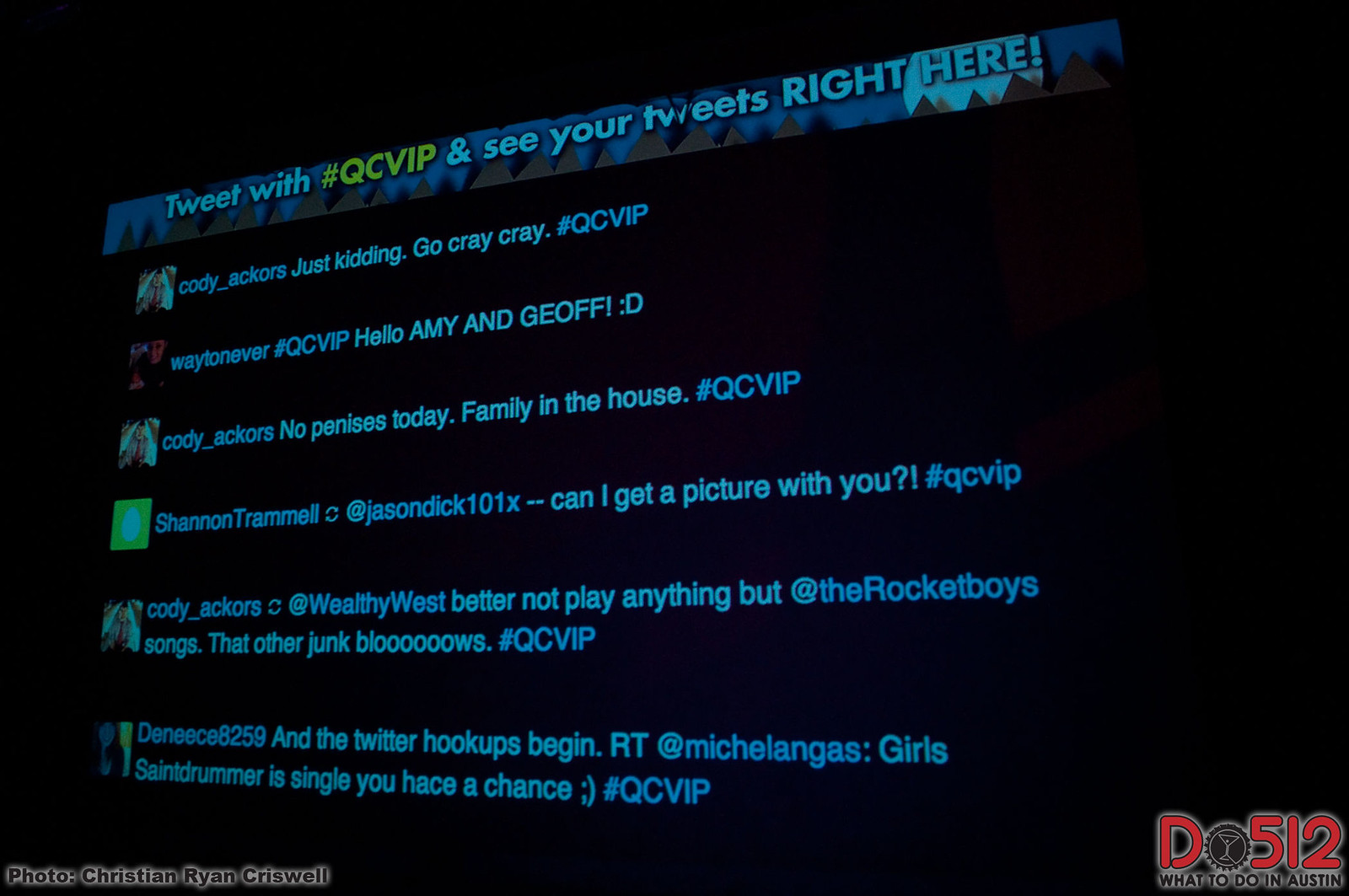The image is a screenshot of a website showcasing live tweets with the hashtag #QCVIP against a predominantly black background. At the top, a blue banner with grey triangles resembling a stylized forest, complete with a sun or moon at the right, invites users to "Tweet with hashtag #QCVIP and see your tweets right here." Below, six tweets are displayed in white sans-serif text that appears blue due to the image's coloring. 

Prominent tweets include Cody Ackers (miswritten as "Cody underscore actors" in previous captions), who humorously tweets, "Just kidding, go cray cray #QCVIP" and "No penises today, family in the house #QCVIP". Weyton Ever greets with, "Hello Amy and Jeff :)" using the same hashtag. Shannon Trammell requests a photo with "Jason Dick 101X," and Cody Ackers again insists, "At Wealthy West, better not play anything but at the Rocket Boys songs, that other junk blows #QCVIP." Denise8259 announces, "And the Twitter hookups begin, RT at Michelangelo's Girls St. John Mary's single, you'll has a chance,” signing off with a winky emoji.

A watermark on the lower right corner reads "D512 What to do in Austin" in red text, while the lower left corner credits the photo to Christian Ryan Criswell. The tweets are accompanied by small profile images of the senders on the left.